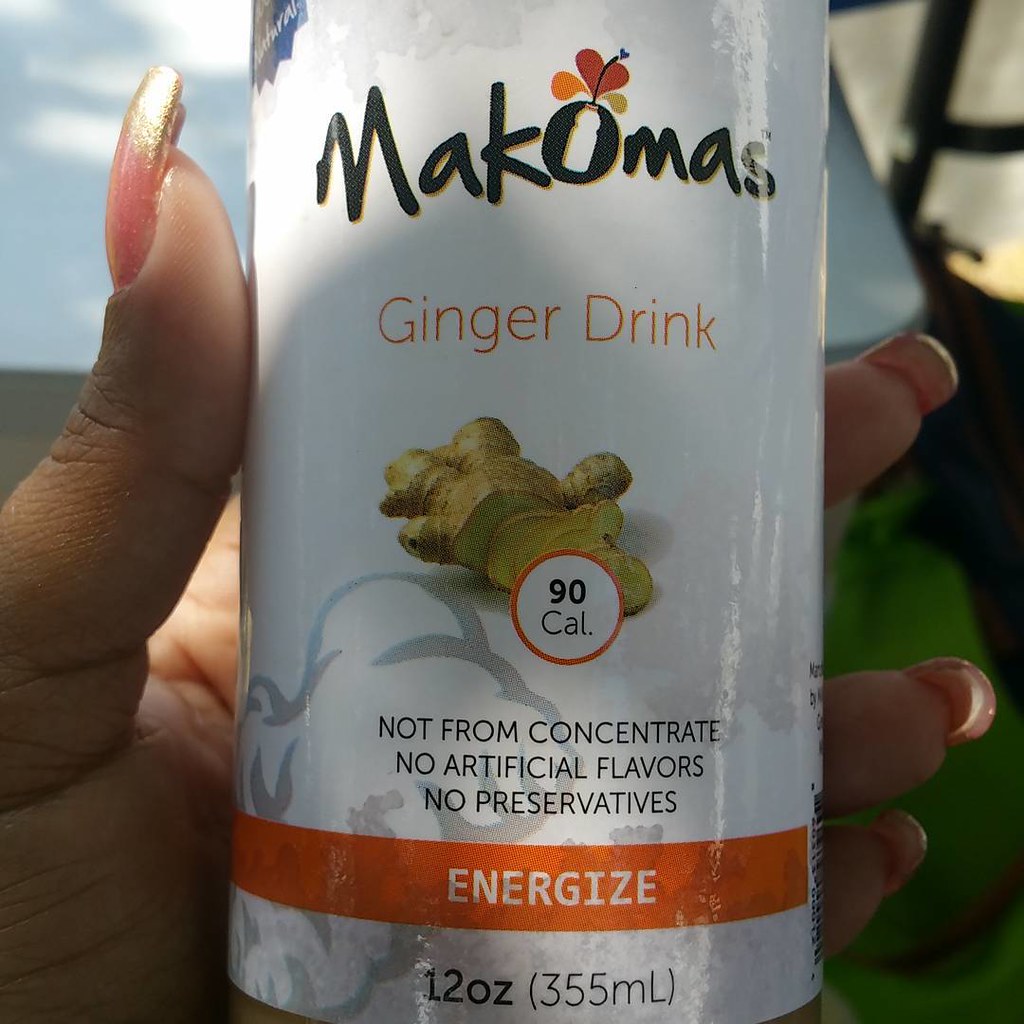A vibrant, close-up shot captures a woman's left hand elegantly holding a can of Macomas Ginger Drink. Her long nails, painted in a glamorous pink with gold tips, add a touch of sophistication. The can, prominently featured, is decorated in white, orange, and green hues with enticing text and graphics. At the top, "Macomas" is inscribed, followed by "Ginger Drink" under a detailed illustration of ginger root adorned with a circle proclaiming "90 CAL." The bottom of the can highlights its natural qualities: "Not from concentrate, no artificial flavors, no preservatives," all above an orange strip emblazoned with "Energize." Below this, the can’s volume is marked as "12 ounces, 355 milliliters." The shadows falling over the can suggest the image was taken outdoors, bathed in sunlight that creates striking highlights and shadows, enhancing the vivid colors likely accentuated through photo editing.